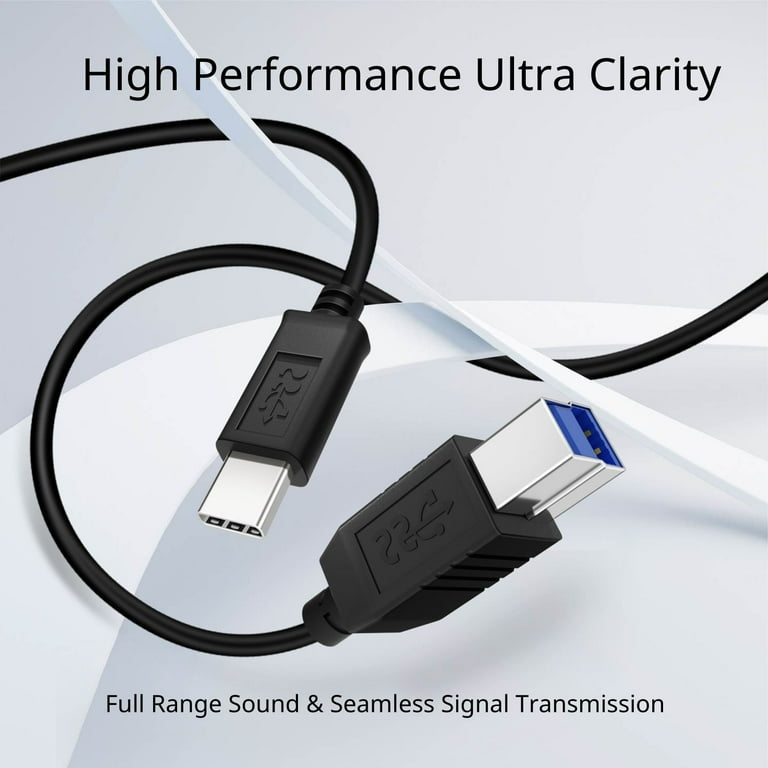The image showcases a tangle of sleek black cables set against a nuanced gray background. Dominating the scene is a USB Type-C to USB Type-B cable that enters from the left side of the frame. The USB Type-C connector, positioned on the left, leads a coiled path, first intertwining with a white ribbon, and then continuing off-screen. From the right, another similar black cable intrudes, snaking underneath and above the white ribbon to converge near the image's center where the silver, blue-interior USB Type-B port is prominently displayed. Both cables thread and loop around the central white line, creating an intricate, almost artistic, crisscross pattern. Text is positioned at the top and bottom of the square image canvas; the top text reads "High-performance, ultra-clarity" in bold black font, while the bottom is slightly smaller, stating "Full-range sound and seamless signal transmission," highlighting the capabilities and quality of the cables.